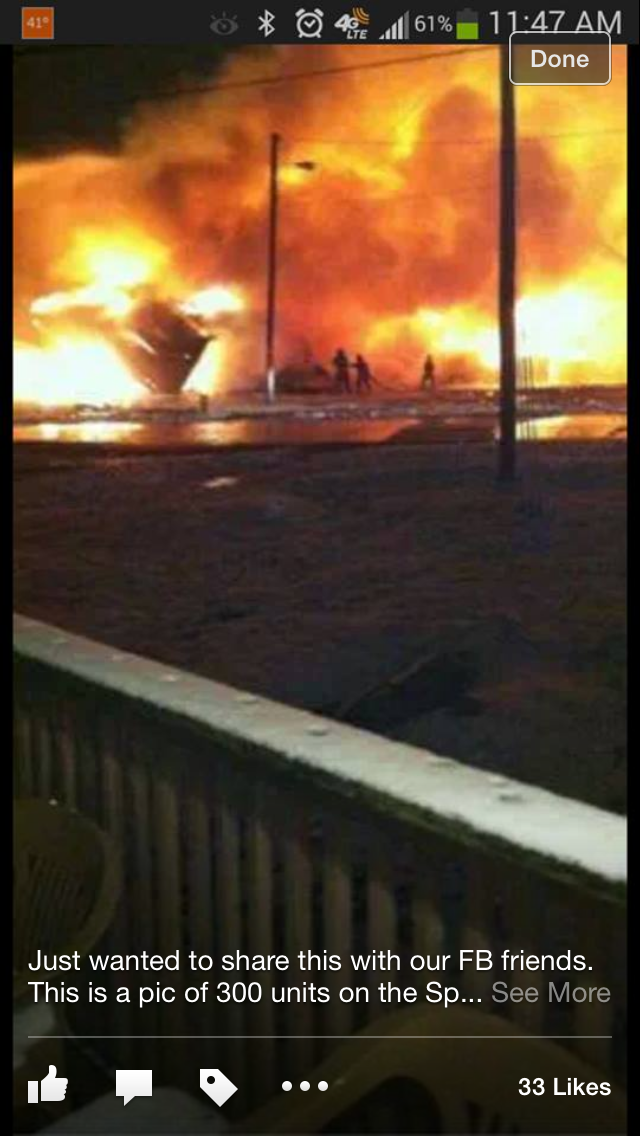The image is a screenshot of a Facebook post displayed on a cell phone, as indicated by the black border at the top with icons, a percent meter, and the time showing 11:47. The photo within the post captures an intense fire scene from the vantage point of the front porch of a house. In the foreground, you can see a wooden fence, two plastic chairs, and part of a railing. The background reveals a raging fire with three firemen actively battling the flames using a hose. To the right of the fire, a couple of people and large utility poles are visible, with a street and dirt ground beneath them. The caption beneath the photo reads: "Just wanted to share this with our FB friends. This is a pic of 300 units on the SP..." followed by "See More" for further text. Below the caption are engagement icons: a thumbs-up for liking, a comment bubble, a tag option, and three dots for more features. The post has garnered 33 likes.